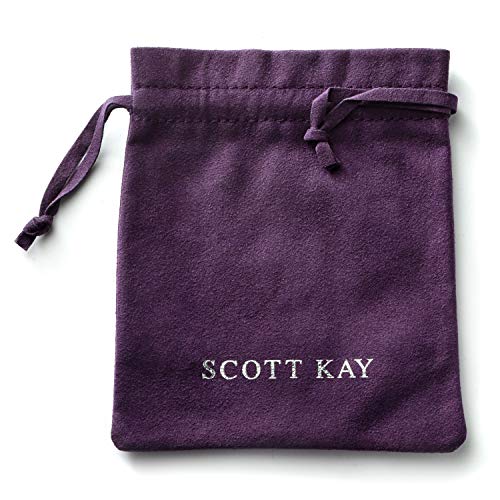This close-up photograph features a dark purple, suede-like jewelry pouch against a completely white background. The rectangular pouch is open at the top, showcasing two knotted drawstrings extending from its sides, designed for cinching it shut. The material of the pouch appears richly textured, with stitching details visible near the top. At the bottom of the pouch, silver screen-printed lettering spells out "SCOTT K" in capital letters. Light from the upper right creates gentle shadows on the front and underneath the pouch, highlighting its slightly bent and curved edges at the bottom. This elegant storage bag, in a deep plum hue, displays a hint of wear, evidenced by a faint wrinkle, enhancing its velvety, suede-like appearance.